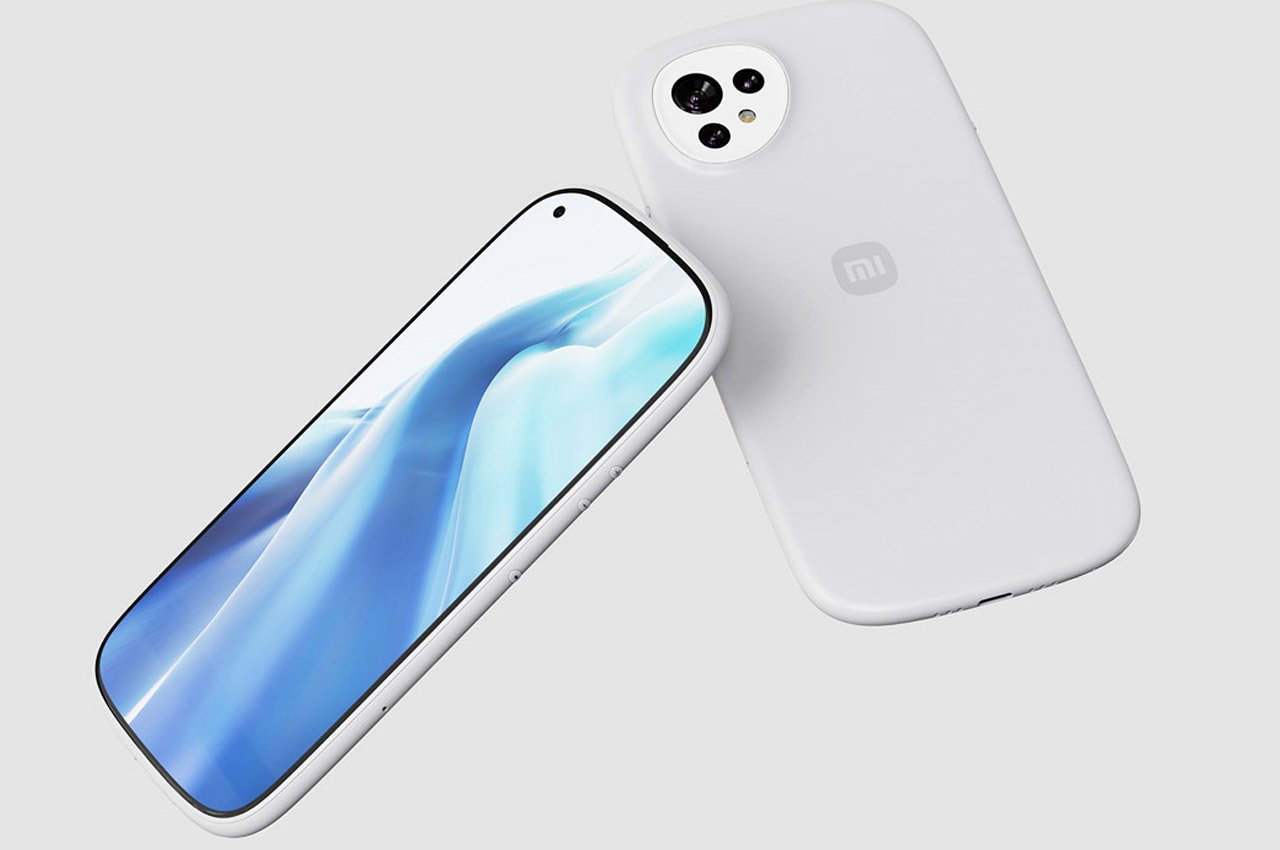The image features two sleek smartphones against a white background, arranged in a landscape orientation. The first phone is upright, displaying a captivating digital screen saver with swirling, abstract waves in varying shades of blue and white, giving a watery impression. This phone's front camera is subtly located in the upper left-hand corner. Adjacent to this, the second phone is positioned at an angle, showcasing its back. It is white or light gray in color, prominently featuring a gray "MI" logo in the center. The upper left corner of the back displays a sophisticated camera assembly that includes a large lens, two smaller lenses, and a round flash. Together, these phones cast gentle shadows on the background, emphasizing their sleek and modern design, indicative of a high-end smartphone advertisement.